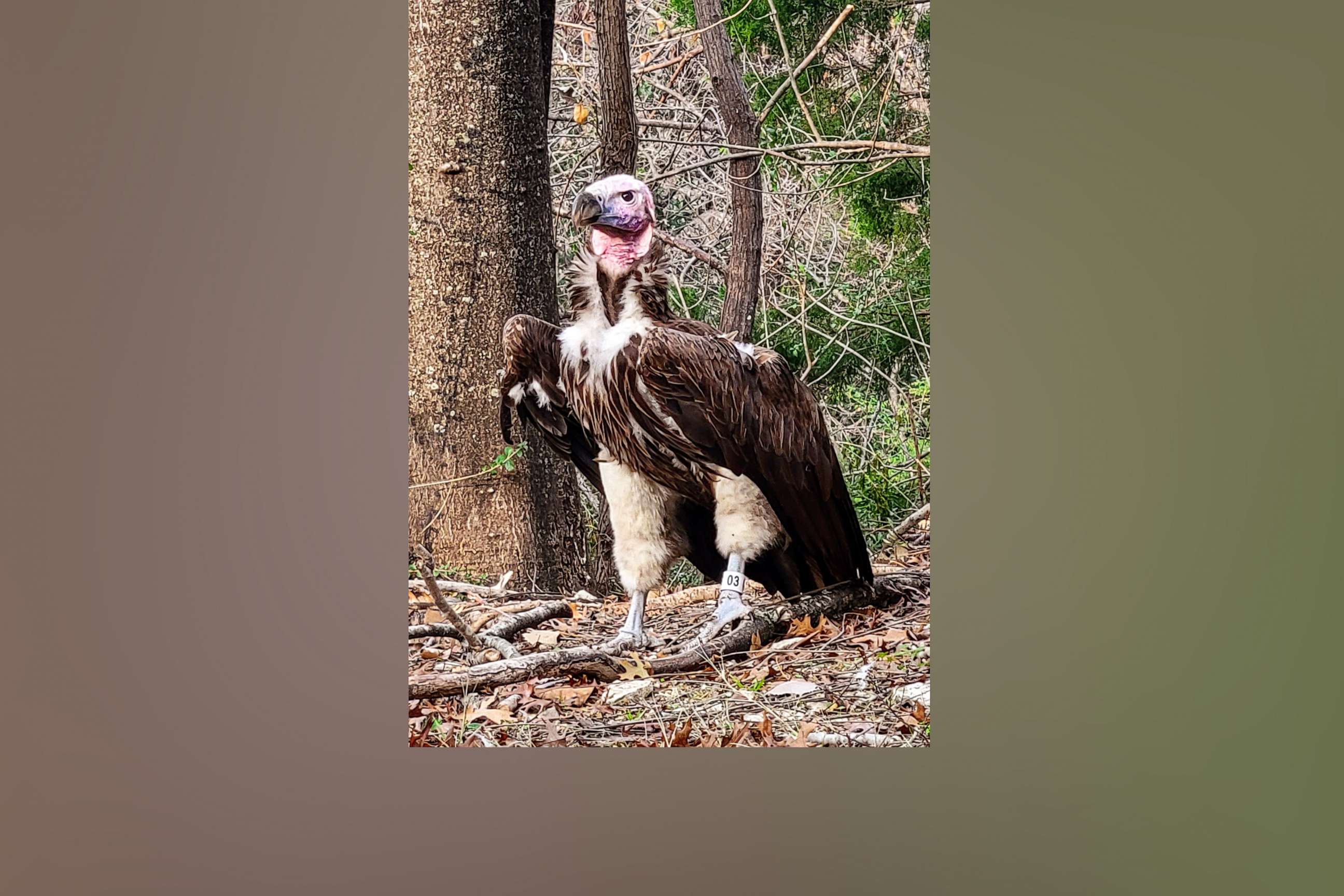This vertical photograph features a buzzard standing prominently in the center of a forested area. The bird is positioned on the forest floor amidst a scattering of leaves, broken branches, and dirt. To its right stands a large tree, with the trunks of several smaller trees visible behind it, and a greenish area suggesting foliage in the background. The buzzard has distinct, fluffy beige feathers that cover its legs, and a tag on its left leg marked "03" in black font on a white label. Its body is coated with dark brown feathers, and its wings are slightly tucked back. The bird's chest shows some white feathers, and it has a long neck with a pinkish-reddish tint under its chin, blending into a whitish-beige head. Its eyes are black, though only one is visible, and it boasts a medium-sized dark brown beak. The buzzard is gazing slightly to the left, adding a contemplative element to its stance. The background includes a mix of blurry brown hues and greenery, enhancing the woodland setting of this detailed and evocative wildlife image.